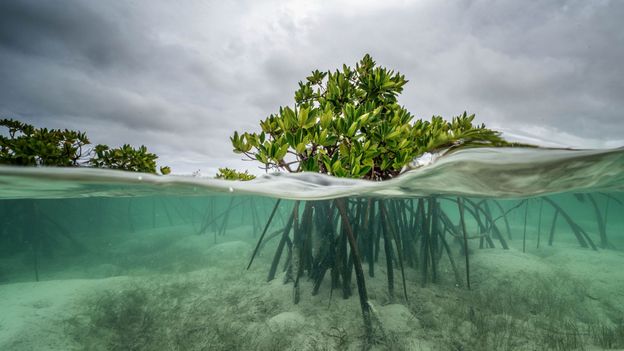The color photograph captures a split-view scene, showcasing an aquatic plant, likely a mangrove, both above and below the water's surface. Centrally positioned in the landscape-oriented image, the plant's green leaves extend above the waterline, while its long, brown roots delve into the light, sandy ocean floor below. The ocean floor, sprinkled with beige corals and rocks, stretches across the bottom of the image. A distinct waterline horizontally bisects the photo, highlighting the reflective ripples on the surface. Surrounding the scene, a dark gray sky with scattered white clouds looms overhead, introducing a hint of light from the left side. In the background, flag grasses and trees add depth to the serene environment. A small white rock, slightly right of the center, nestles among the plant's stems at the bottom, enhancing the detailed realism of this tranquil, partially underwater photograph.